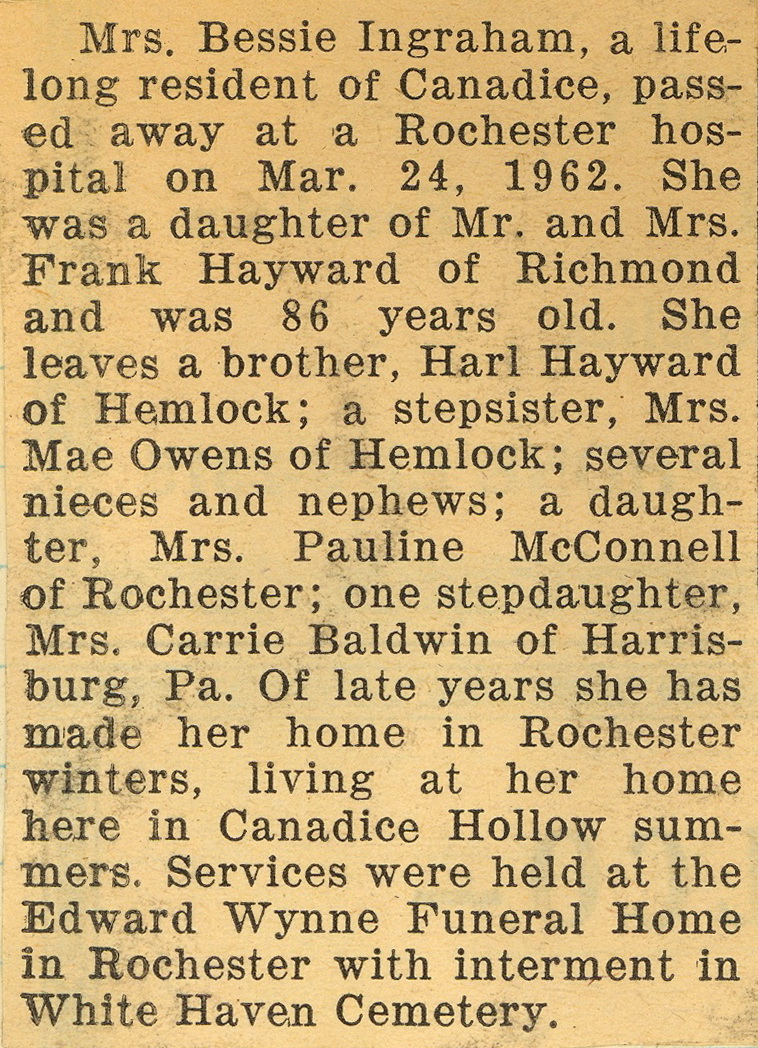This text image portrays an obituary typed on old, browned paper, with a light brown background and black letters. The obituary commemorates Mrs. Bessie Ingraham, a lifelong resident of Canadice, who passed away at a Rochester hospital on March 24, 1962, at the age of 86. She was the daughter of Mr. and Mrs. Frank Hayward of Richmond. Mrs. Ingraham is survived by her brother, Earl Hayward of Hemlock, and her stepsister, Mrs. May Owens of Hemlock, as well as several nieces and nephews. She also leaves behind a daughter, Mrs. Pauline McConnell of Rochester, and a stepdaughter, Mrs. Carrie Baldwin of Harrisburg, Pennsylvania. In her later years, she spent winters in Rochester and summers at her home in Canadice Hollow. The funeral services were conducted at the Edward Vine Funeral Home in Rochester, with burial at Whitehaven Cemetery.